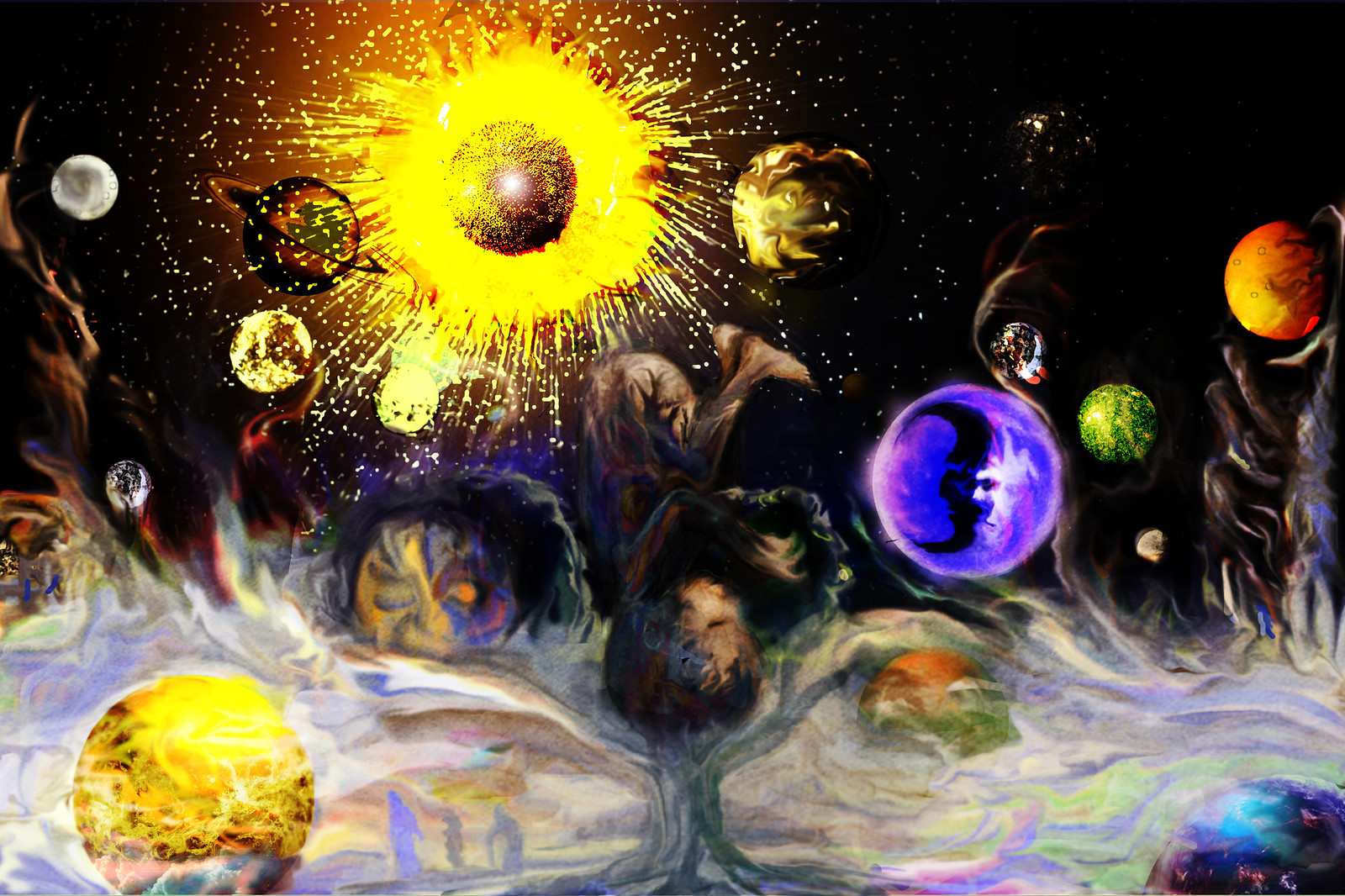This captivating and highly abstract image, potentially a combination of painting and digital art, vividly depicts a cosmic and spiritual scene. The top half of the image features a vast, black space adorned with various celestial bodies. Dominantly, there's a luminous, yellow-orange orb bursting with radiant sparks, suggestive of the sun, framed on its periphery by an intense red glow. Adjacent to this sunburst, Saturn with its iconic rings stands out prominently among other planets and moons. The celestial composition is enhanced by swirling arrays of bright, dynamic colors including gold, blue, purple, green, yellow, and red, crafting a vibrant and artistic tableau.

In the middle of the image, a reddish-brown infant floats upside down, its umbilical cord intricately connected to a tree trunk that emerges from the lower half of the artwork. This central baby figure, with distinguishable legs and arms, symbolizes a profound connection between life and nature. The tree itself branches out from a watercolor-like base, which blends into the lower half of the image that appears almost fiery with swirling patterns. Amidst this fiery, swirling landscape, more planets are dispersed, integrating the celestial theme throughout the entire composition. To the left of the infant, three ghostly figures appear to be walking, adding a mysterious human element to this cosmic and abstract artwork. The fusion of mediums and the rich, detailed imagery make this piece both otherworldly and deeply thought-provoking.